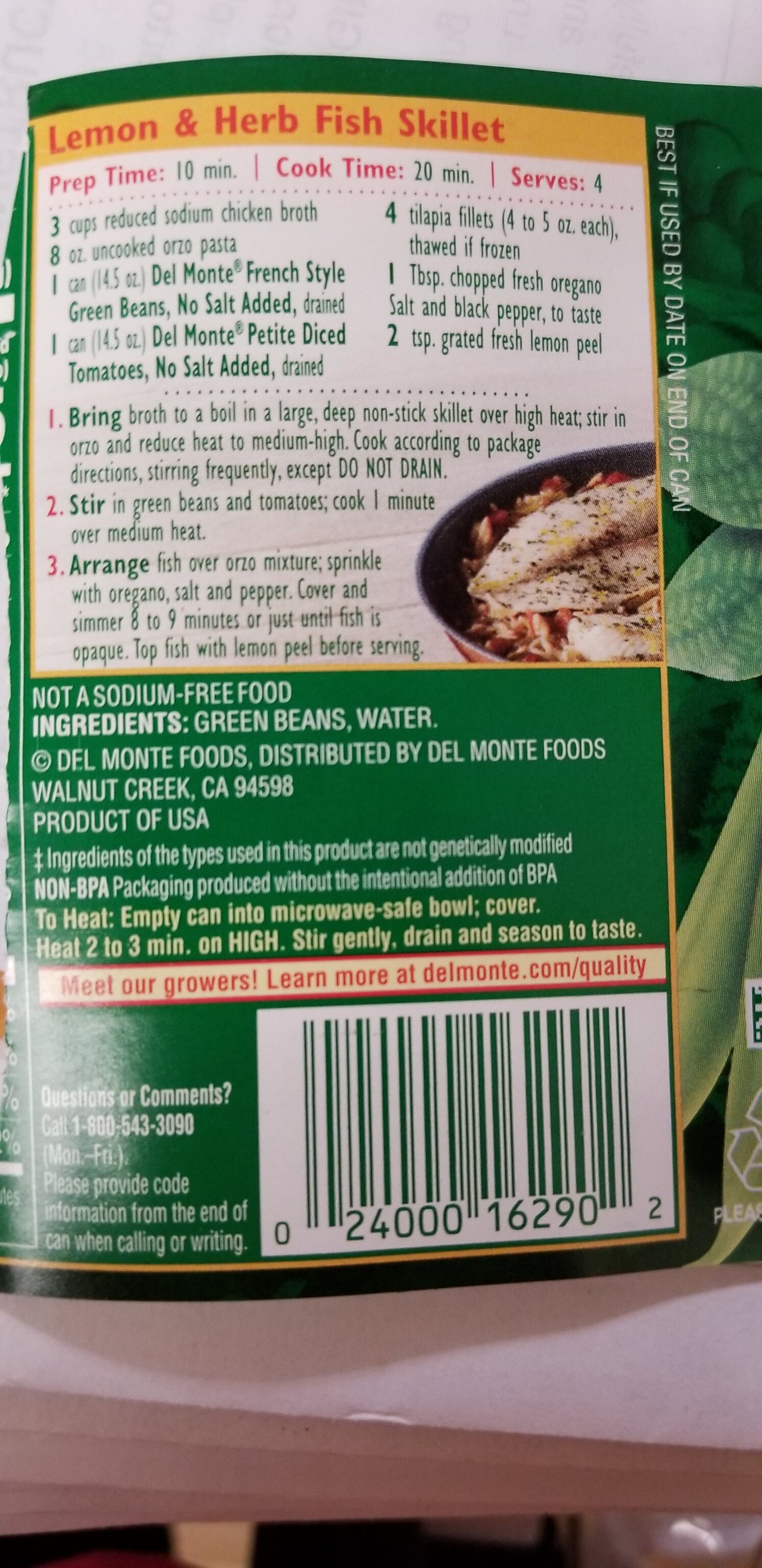This image shows the detailed back label of a green can of Del Monte green beans. The label prominently features a recipe for "Lemon and Herb Fish Skillet" in red text against a white background, with a yellow horizontal band across the top of the recipe section. The recipe details include a prep time of 10 minutes, a cook time of 20 minutes, and it serves 4. It provides step-by-step instructions for preparing the dish, mentioning actions like bringing a pot to boil, using a non-stick skillet over high heat, and arranging fish over a marinade followed by sprinkling with oregano, salt, and pepper. The final step includes topping the fish with lemon peel before serving. Additionally, there's a note that the product is not sodium-free. The can's ingredients are listed as green beans and water. The bottom of the label features a black and white barcode with serial numbers and mentions Del Monte Foods, along with a website for more information: delmonte.com/quality.